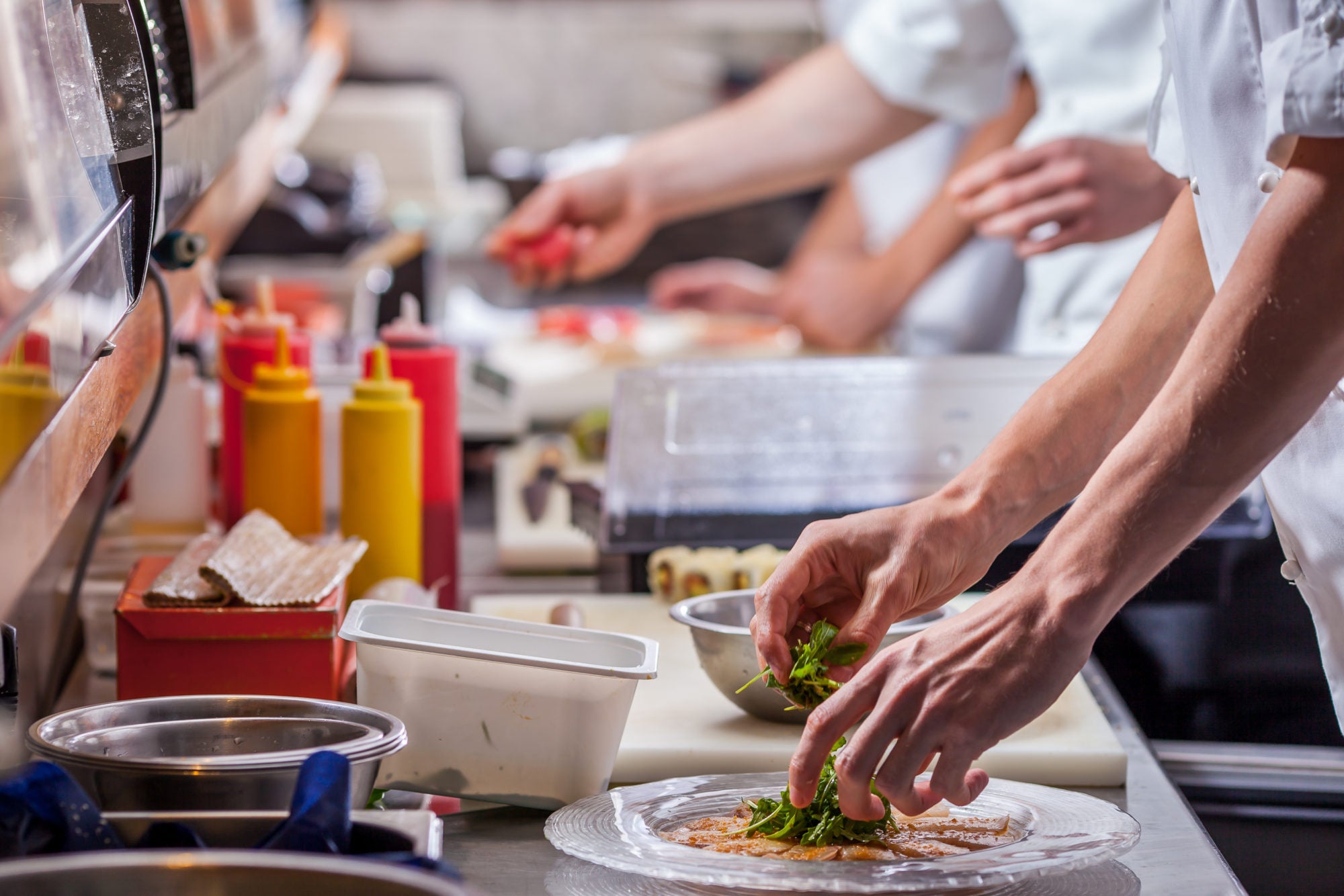In this photograph of a bustling professional kitchen, the countertop is crowded with various food items and kitchen essentials as multiple chefs work diligently to prepare dishes. The countertop features metallic and plastic bowls, condiment bottles with yellow and red hues, and a cutting board. The chefs, identifiable by their traditional white coats, are captured from the chest down with their hands and arms actively engaged in the culinary process. In the foreground, a chef meticulously plates a dish that appears to be carpaccio, skillfully sprinkling mixed greens on top. Nearby, another chef is separated by a large plastic container holding ingredients like lettuce and garnishes. The background is slightly blurred, emphasizing the focused and coordinated effort of this efficient production line as they prepare meals for restaurant patrons. The scene also includes electrical appliances adding to the busy atmosphere of this professional culinary space.